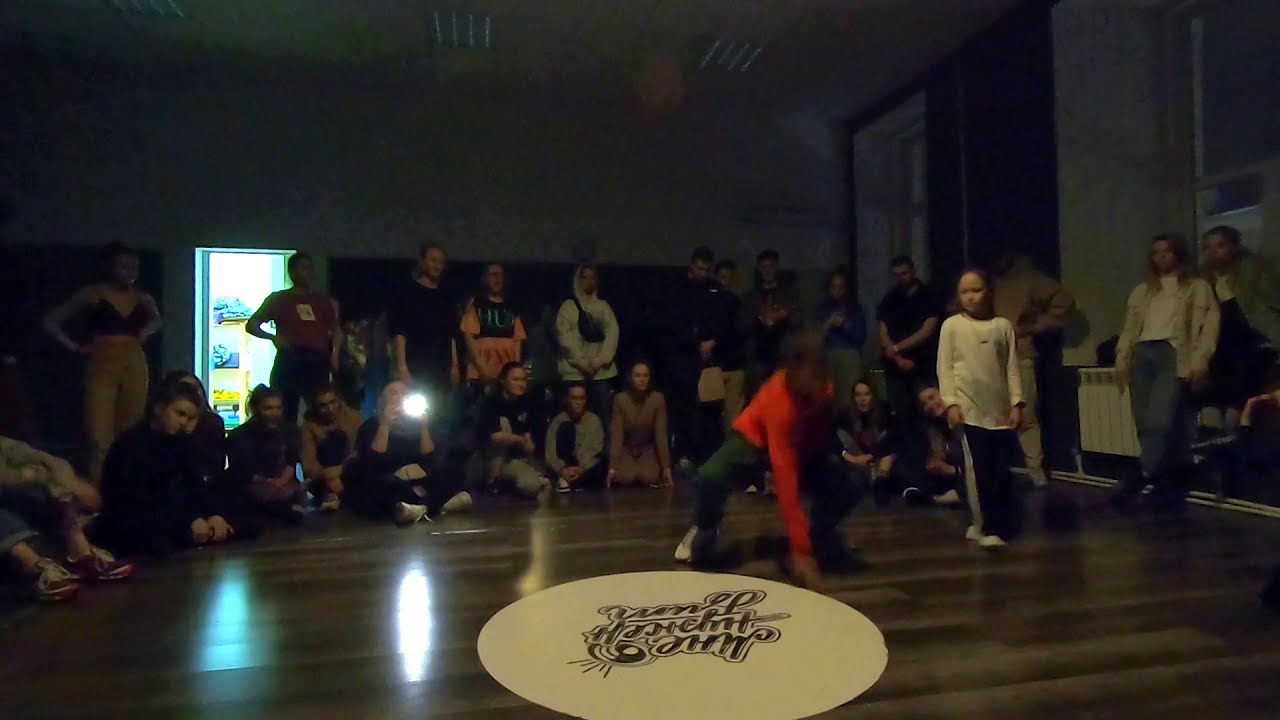In the photograph, a lively scene unfolds in what appears to be a dimly lit dance studio, illuminated by a soft glow from some background lights near the windows. At the center of attention is an individual, possibly a black male, engaging in a dynamic dance move that renders him blurry due to his motion. He is dressed in a vibrant red long-sleeve shirt, which might be a hoodie, paired with dark pants—likely black or green—and white sneakers. This person seems to be breakdancing or performing an energetic routine near a prominent white circle painted on the wooden floor. The circle contains some writing, including the word "June" and possibly "family," though the text is partially obscured and upside down from the photo's angle.

Surrounding the dancer, about 50 onlookers are gathered, forming a ring around the performance space. Some are seated while others stand behind, intently watching the spectacle unfold. The observers vary in age, suggesting a diverse gathering, perhaps a dance class, competition, or team meeting. Adding to the dynamic atmosphere, a young girl is seen walking beside the dancing figure, and someone in the background is capturing the moment with a camera. The overall ambience inside the room is vibrant yet intimate, accentuating the communal spirit of the event.